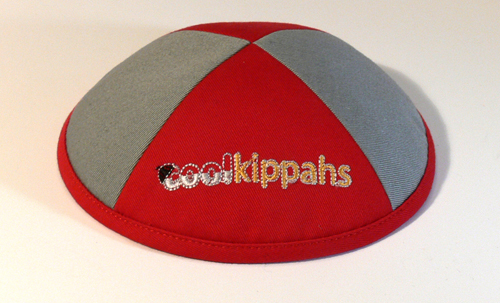This image showcases a children's product, specifically a hat, placed on a cream-colored surface. The hat is circular and sectioned into four parts with alternating grey and red segments. The central red part features the logo "Kool Kappas," with "Kool" written in white and red fonts and a small black hat design atop the "K." The word "Kappas" is woven in yellow fonts. The hat appears new and pristine, illuminated by professional lighting that casts shadows on both the left and right sides. The overall photograph is clear and detailed, highlighting the hat's vibrant colors and clean design.